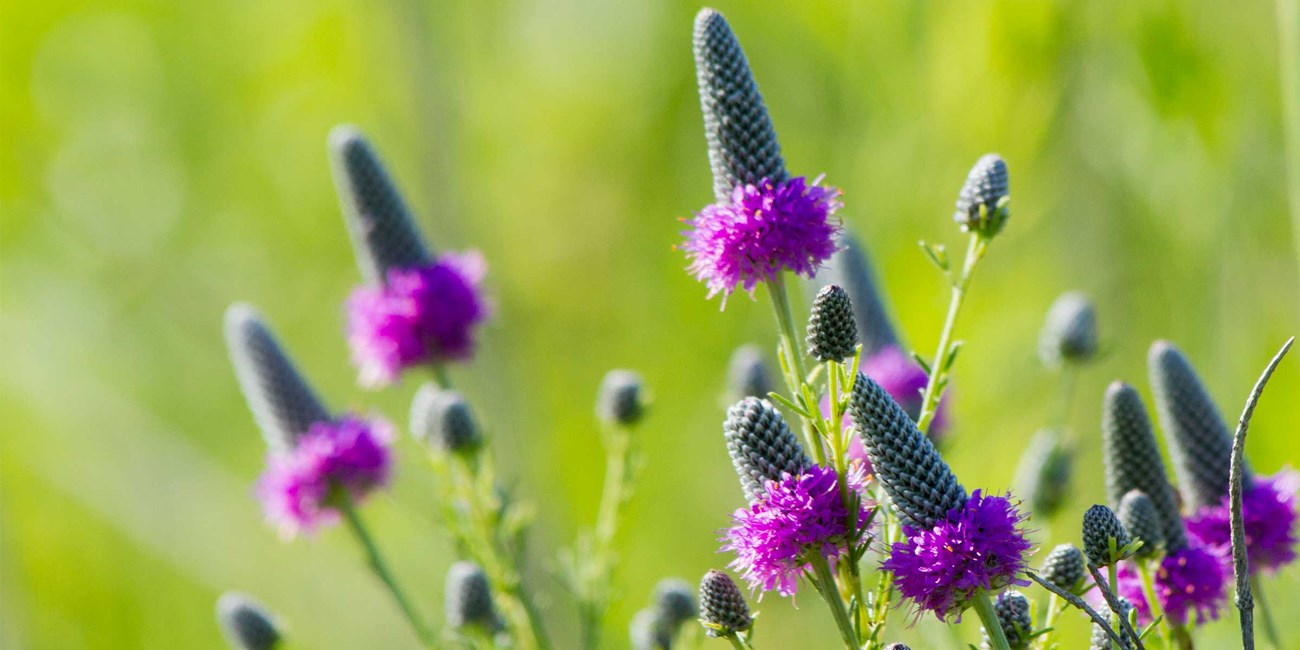The image is a close-up of numerous purple flowers, predominantly featured from the bottom right to the left side of the frame. The emphasis is on a few flowers in the foreground, with blurred versions of the same flowers in the background, creating a depth of field effect. Each flower is supported by tall, green stems that branch out towards the top. The flowers exhibit fluffy purple petals reminiscent of cornflowers or bachelor's buttons, surrounding elongated green cone-shaped centers that resemble pinecones or raspberries. Some flowers only have the cone visible, without any petals. The background features a soft blur of various shades of green, with hints of yellow and white, possibly suggesting grass or other flora, further enhancing the focus on the vividly detailed flowers in the foreground.